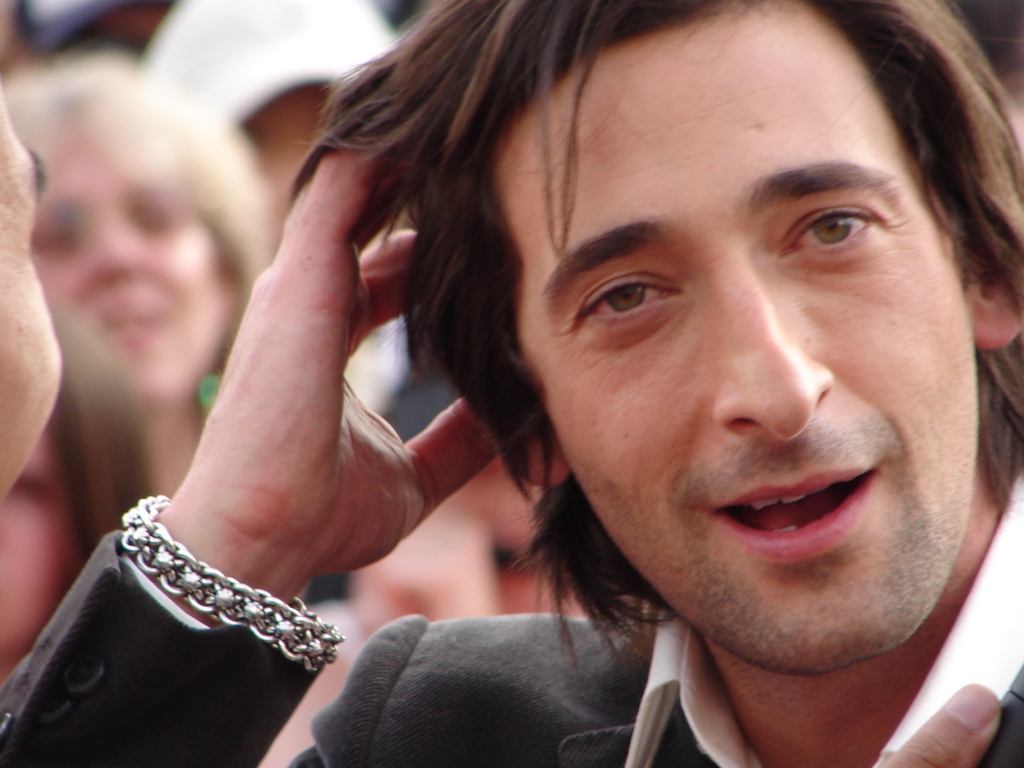This image captures a white male actor, known for his prominent five o'clock shadow, beard, and mustache, and distinguished by his shaggy dark brunette hair that falls just past his ears. He has expressive hazel eyes and appears to be in mid-conversation, his mouth open slightly revealing his teeth and tongue, almost as if caught in a partial smile suggesting he is in a good mood. Clad in a sophisticated gray suit paired with a white button-down collared shirt, he accessorizes with a distinctive silver link bracelet on his left wrist. His left hand touches the left side of his head near his ear, with his head slightly tilted. The photograph is taken on a red carpet, with a crowd of men and women visible in the blurred background, adding to the atmosphere of an event or premiere.